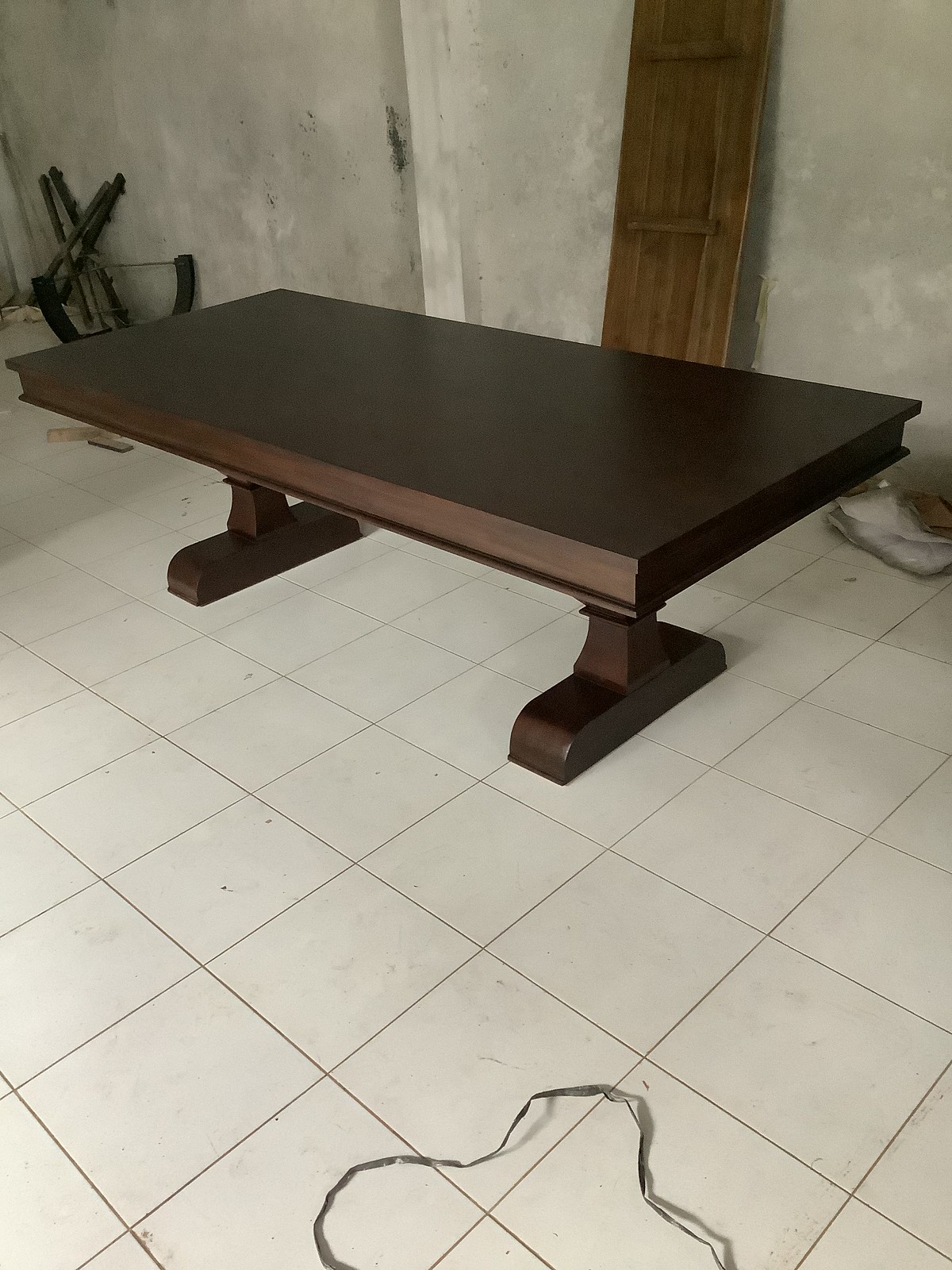This color photograph appears to be taken inside a basement, characterized by a dirty, possibly moldy concrete wall in the background. A large, brown rectangular wooden plank is propped vertically against the right side of the wall. In the center of the room, there is a dark, rich walnut-colored wooden table, reminiscent of an old-fashioned library table. This table is uniquely designed with only two columnar legs, each terminating in a long base for stability. The table's dark wood contrasts strikingly with the tiled floor beneath it, which is composed of small, white ceramic squares. Near the bottom middle of the image, a piece of gray wiring or perhaps a ribbony plastic object, resembling a rope, is laid out on the floor. In the background, near the upper edge of the photograph, there seems to be a white fabric curtain, adding to the overall disarray of the scene.